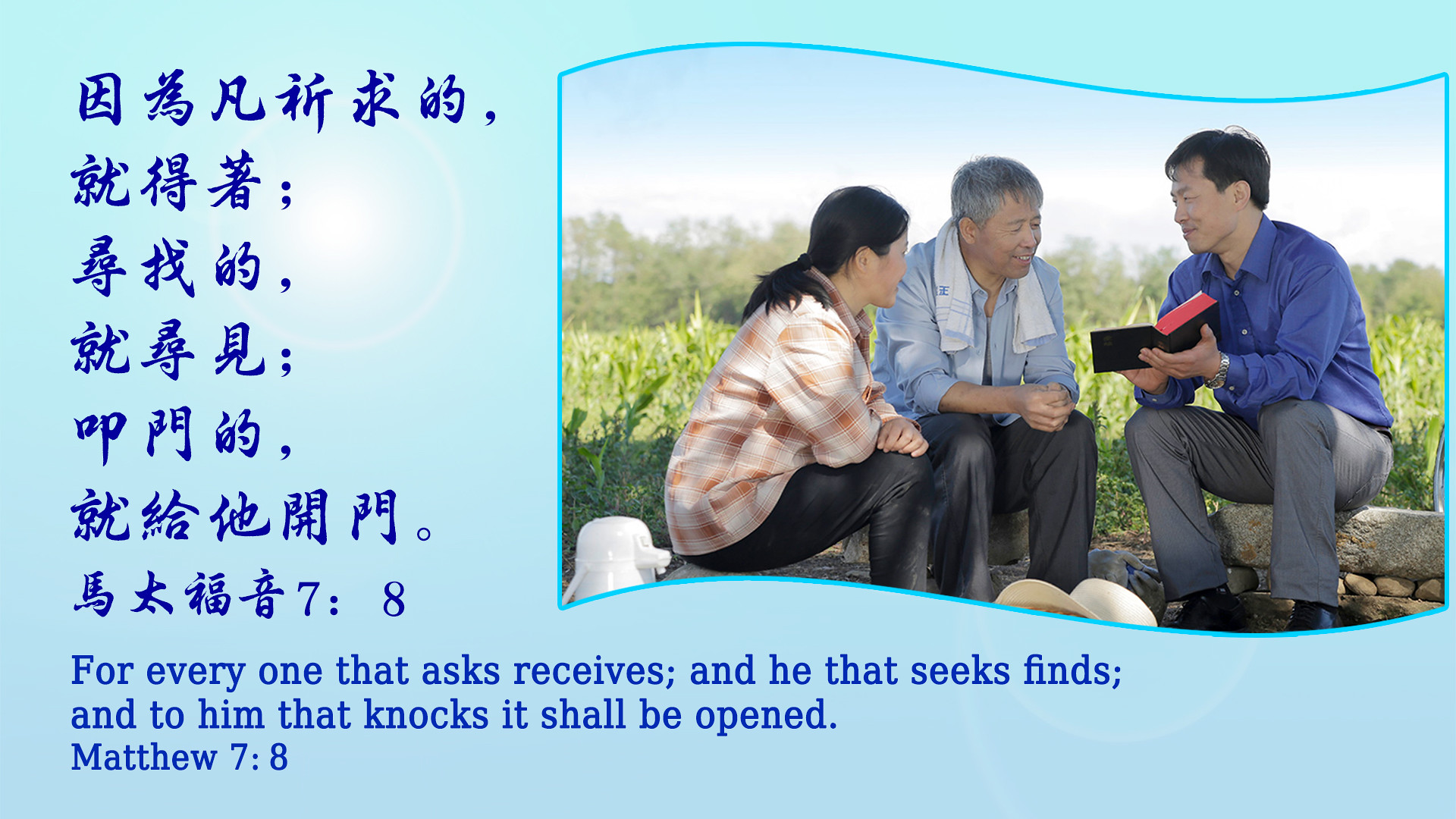The flyer features a light blue background, accented with a few touches of white, and contains both Chinese characters and an English translation of a religious proverb. The Chinese text runs vertically almost the entire height of the left side of the flyer and ends with the numbers "7" and "8". At the bottom, the text “For everyone that asks, receives; and he that seeks, finds; and to him that knocks, it shall be opened. Matthew 7:8” is written in dark blue font. 

On the right side of the flyer is an image resembling a flag, depicting three people outdoors, sitting on what appears to be a constructed stone seating area. The man on the right, dressed in a blue shirt, is holding an open, thick book, presumed to be a Bible, showing it to the other two individuals. The second man, to his left, is wearing a light blue shirt, and a woman with long hair flowing past her shoulders is next to him. All three are engaged in what looks like a thoughtful discussion, deeply focused on the content of the book. The scene is set in a natural environment, suggesting an informal yet meaningful interaction around the shared reading.